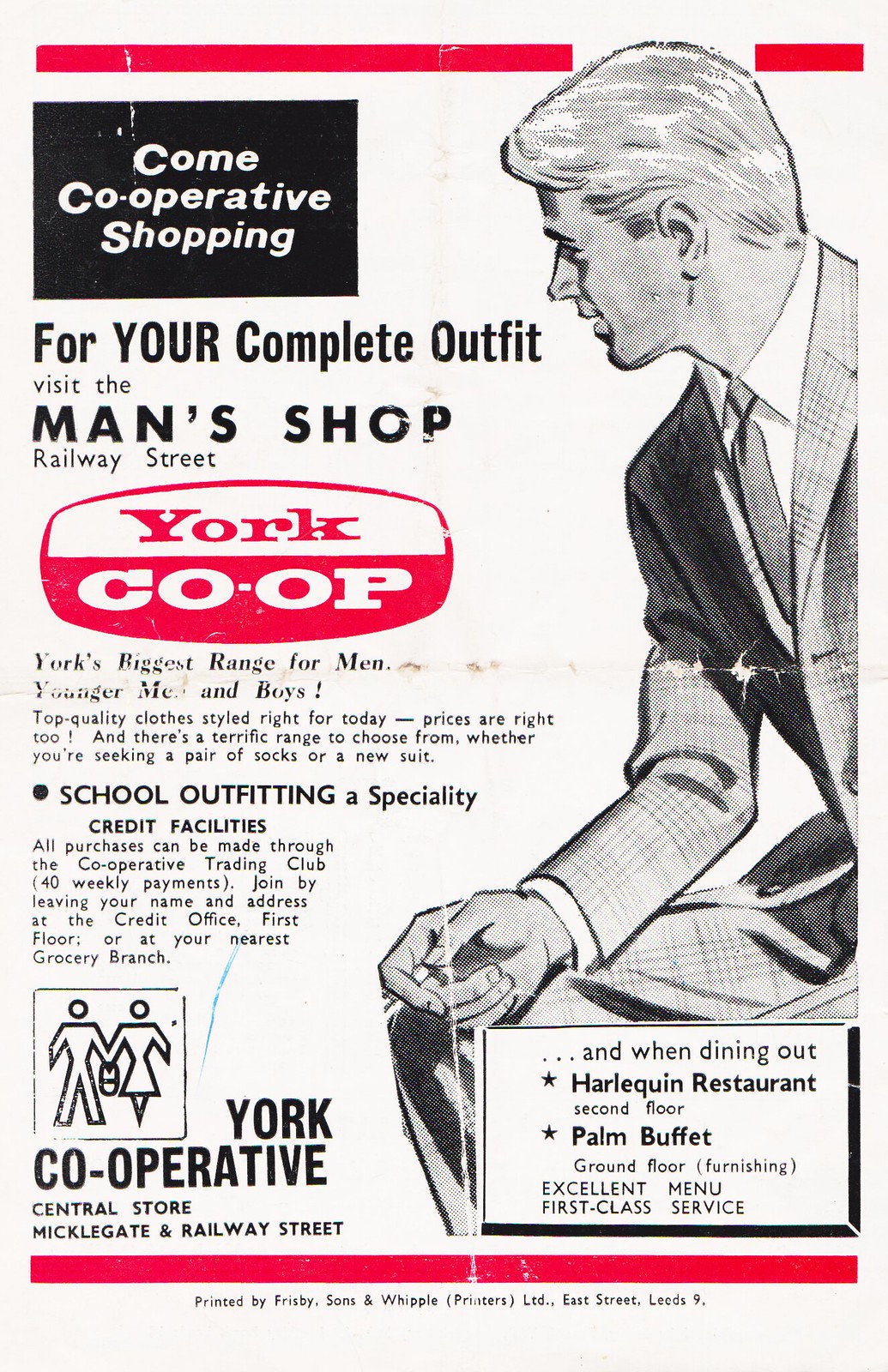This photograph features a vintage-style poster with a white background. On the right side of the poster, there is a detailed drawing of a man seated, dressed in a formal outfit consisting of a coat, tie, and trousers. The poster's text is predominantly in black, save for the words "York Co-op," which are highlighted in a different color for prominence.

On the left side of the poster, the top section reads, "Come Cooperative Shopping," inviting customers to explore the offerings. Below this, it encourages visitors to "visit the Men's Shoppe, Railway Street, York Co-op" for a complete outfit. Beneath this heading, additional information is provided in smaller text.

In the bottom left corner, the text specifies the locations with addresses reading, "York Co-op, Central Store, Meikle Gate, and Railway Street." The bottom right corner of the poster promotes dining options available within the establishment: "and when dining out, Hardlequin Restaurant, Second Floor, Farm Buffet, Ground Floor, Furnishing, Excellent Menu, First Class Service."

Adding to the visual appeal, there are pink horizontal strips at both the top and bottom of the poster, creating a striking frame for the advertisement.